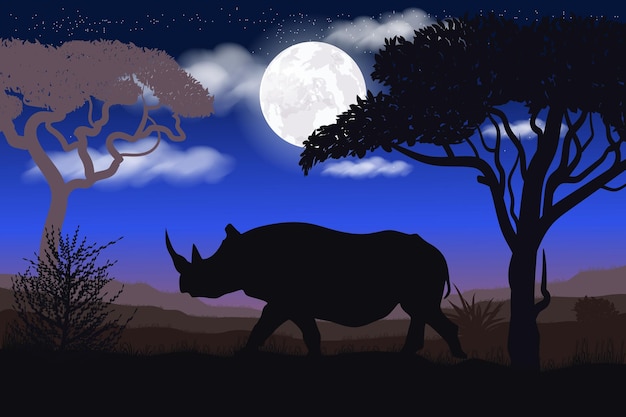This captivating digital painting presents a serene nighttime African scene, framed within a rectangular shape approximately four to five inches wide and three inches high. Dominating the center, a black silhouetted rhinoceros trudges from right to left, highlighting its recognizable horn, legs, and snout, against a plain black ground with patches of grass poking through. To the far right, the silhouette of a tree with intricate branches and leaves stretches to the top right-hand corner. A small bush decorates the ground to the left of the rhino while another tree, displaying a dark brown silhouette, stands on the far left.

The background reveals a masterful gradation of colors: transitioning from a deep black at the base, through varying shades of brown from dark to light, finally meeting a thin purple horizon line. The sky above unfolds into a calm expanse of gradient blues, accented by scattered white clouds. A brilliant full moon radiates at the center, detailed with intricate shapes and patterns, casting a gentle glow over the scene, while delicate white stars sprinkle the uppermost black sky. This tranquil portrayal captures the mystical essence of an African night, blending detailed silhouettes with a calming, multi-layered backdrop.